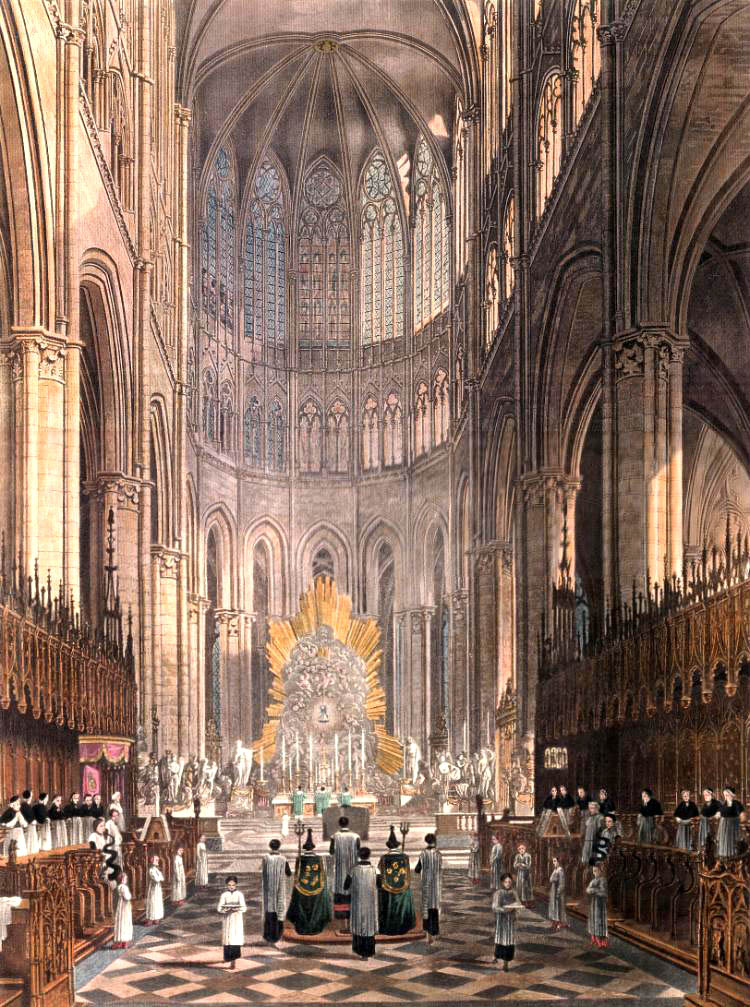The image depicts an ornate, historical painting of a cathedral interior during a ceremonial event. The grand, curved ceiling, supported by towering stone arches, emphasizes the building's immense height. On both sides of the cathedral, observers in uniform attire are perched on ledges. The marble floor, with its intricate X-pattern of black, tan, and gold tiles, adds to the opulence of the scene. Dominating the center of the background is a striking gold and grayish-brown monument, resembling sunbursts, which stands behind a prominent altar. The cathedral’s towering stained glass windows begin halfway up and extend to the top, casting colorful light across the space. Men and women in long robes of white, gray, green, and black walk up and down the central corridor, some carrying staffs or spears, contributing to the solemnity of the ceremony. Rich pink drapes hang on the right side, further indicating the ritualistic importance of the event.